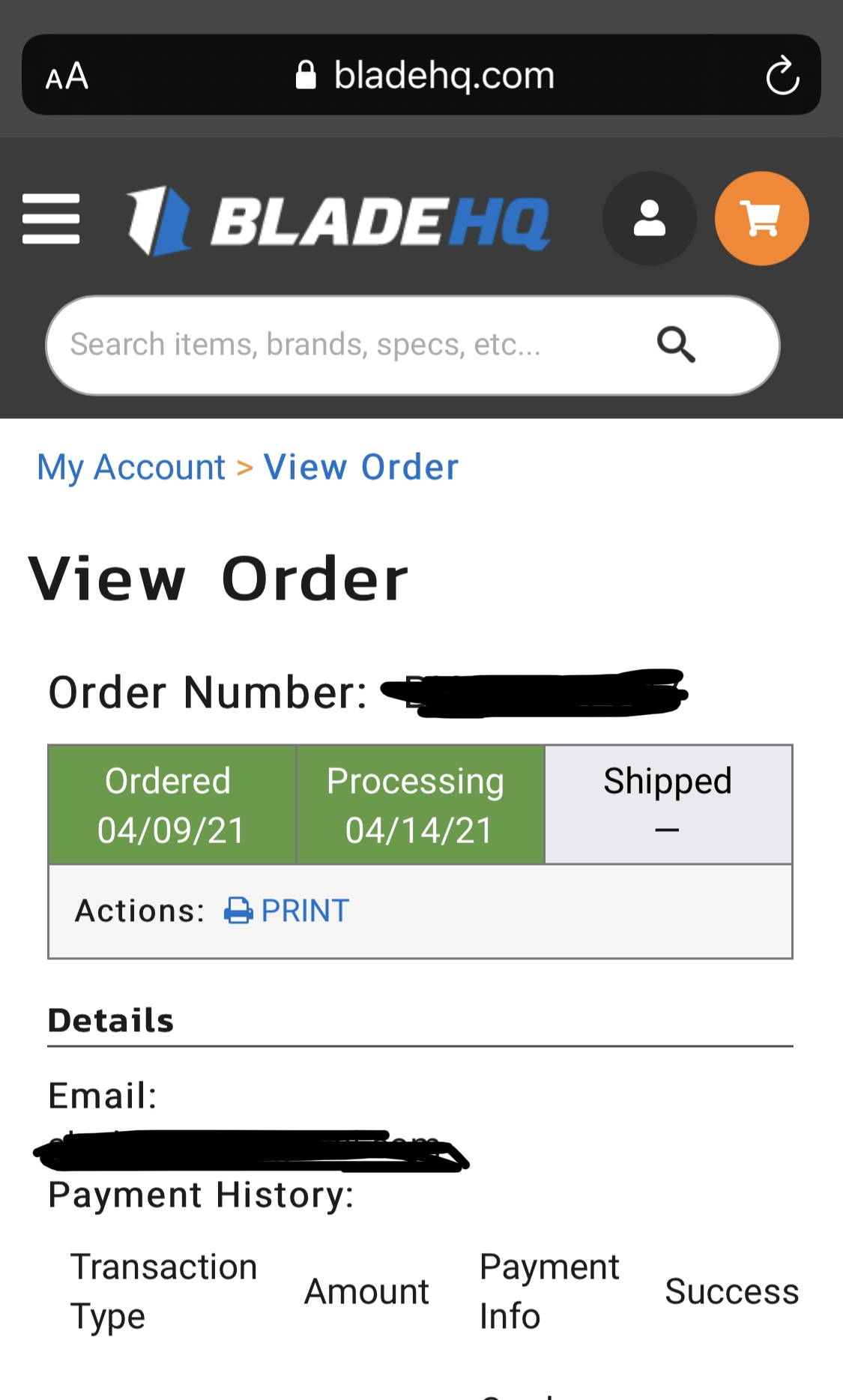Screenshot of an order details page on Blade HQ's website. The top section features the Blade HQ logo, a search bar with the placeholder text "Search brands, specs, etc.," and a navigation menu with options such as "My Account," "View Order," and "View Order (Order Number Redacted)." The order details indicate that the order was placed on April 9, 2021, and is marked as "Processing" since April 14, 2021, but it has not yet been shipped. 

The page includes various sections displaying information relevant to the order, including email, which is redacted for privacy, and payment history, which lists transaction type, amount, payment info, and status marked as "Success." There is also an icon for printing the order details. The background is plain white without any additional design elements. The screenshot likely highlights the customer's dissatisfaction due to the lengthy processing time, as the order remains unshipped after an extended period.